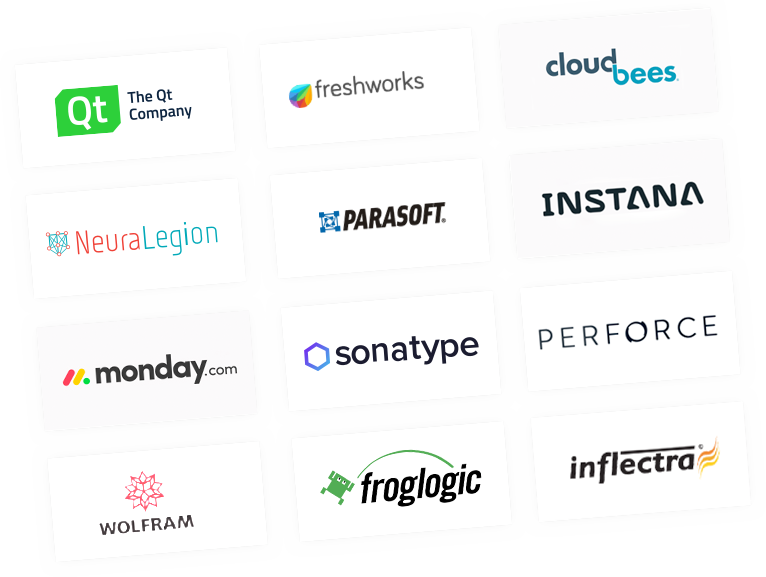Sure, here's a detailed and cleaned-up caption:

"In this image, there are multiple company logos neatly organized within white boxes, each outlined in gray. These boxes are arranged in a grid formation with three columns. Each column contains three or four company names, all of which are tilted slightly towards the upper right. Starting from the top right, the first logo is for the QT company, featuring a green symbol with 'QT' in white. Below it is the Freshworks logo, which displays a multicolored teardrop shape. Next is CloudBees, showcased in a blue color scheme, followed by NeuroLegion, which features blue lines connected by red circles. Perisoft's logo appears next, highlighted by multiple blue squares. Continuing down, the logos of Instana, Monday.com (marked with red, yellow, and green lines), Sonatype, and Perforce are shown. The second column features the Wolfram logo, recognized by its distinctive red flower design, followed by Froglogic’s logo, depicting a green character jumping. The last company, Inflectra, completes the set of prominently displayed logos."